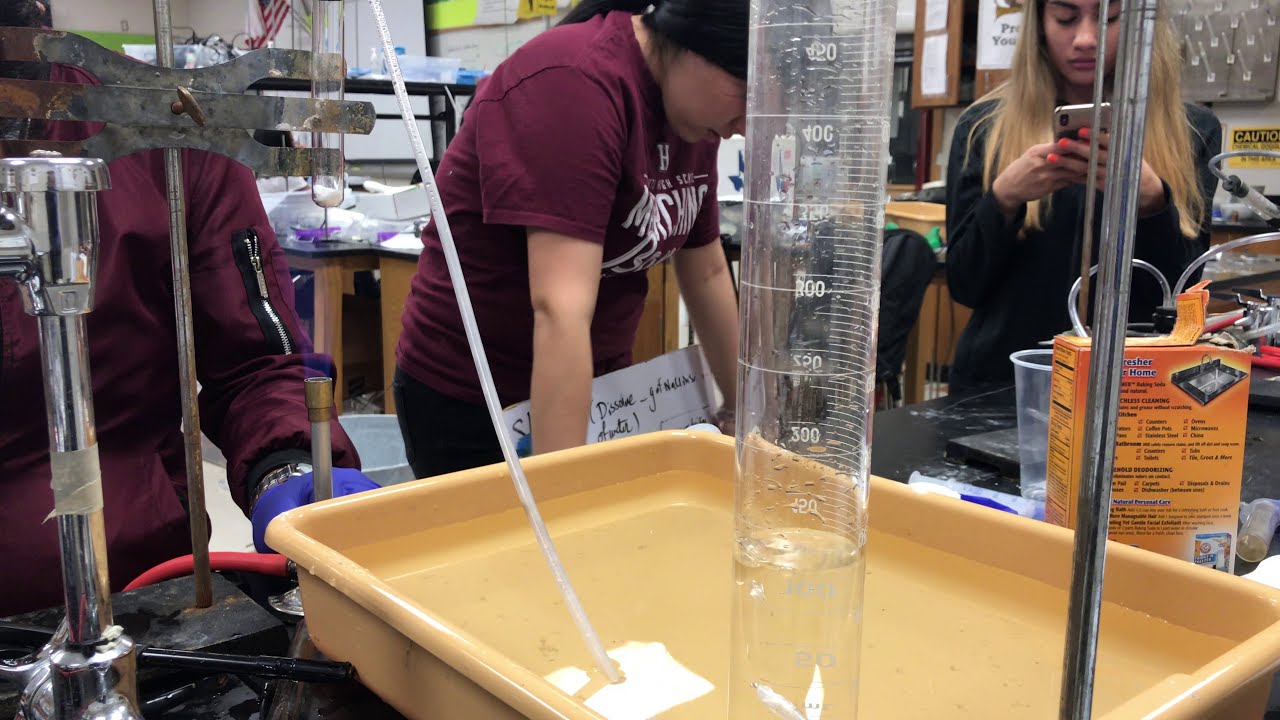The photograph captures a high school science lab bustling with activity centered around a science experiment. Three students are in focus: two wearing maroon tops and a blonde girl in a black long-sleeved shirt with neon orange nails, who is distracted by her phone. The girl with dark hair, tied in a ponytail, and wearing a maroon short-sleeved t-shirt, is leaning over a black table and examining materials, including a tan rectangular container filled with water, a clear test tube, and an open box of Arm & Hammer baking soda. Another figure in a maroon long-sleeved shirt and purple gloves, positioned towards the right side, is handling a test tube over a Bunsen burner. Surrounding the students are various lab equipment, including beakers with measurement markings, plastic trays, and a small plastic cup, contributing to the detailed and dynamic scene.